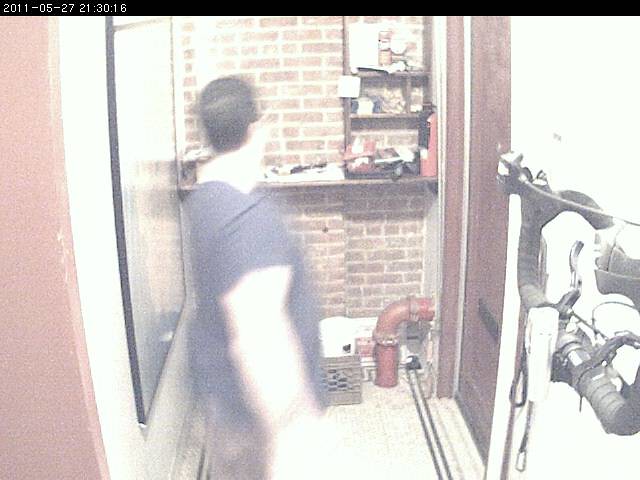This image, captured by a grainy security camera with a black border and a date and time stamp in the upper left corner, shows a narrow hallway or room with a red brick wall at the back. The floor is tiled with a black or blue border. A heavy-set man with black hair, wearing a short-sleeved blue shirt, partly gray or indistinguishable pants, is seen standing at an angle near the left wall, facing away from the camera towards the door on the right. The man appears blurry, particularly around the arms and neck. Along the brick wall at the back, there's a mounted wooden shelf cluttered with several items and a tray on the top right portion. Under the shelf, there’s a small red pipe extending from the right wall into the floor. Mounted on the right wall is a system of red and black pipes and a doorway, possibly accompanied by bicycle handles and some sort of wall art or portrait near the man.